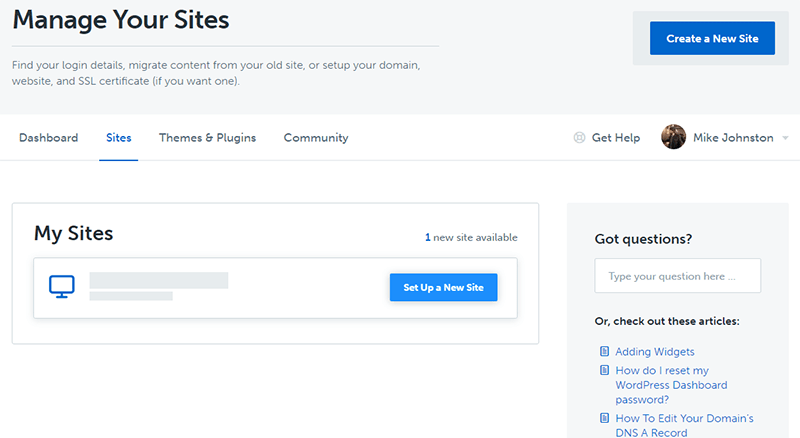The image is a screenshot of a website management interface. 

1. **Header Section**:
    - At the top-left corner, the text "Manage Your Sites" is prominently displayed.
    - At the top-right corner, a blue rectangular button with white text reads "Create a New Site."

2. **Main Content Area**:
    - Directly beneath "Manage Your Sites," instructions for managing site essentials are provided: "Find your login details, migrate content from your old site or set up your domain, website, and SSL certificate if you want one."

3. **Navigation Menu**:
    - There are four main categories listed horizontally:
        - **Dashboard**: This is the first category.
        - **Sites**: Currently selected, this category is highlighted in blue.
        - **Themes and Plugins**: This is the third category.
        - **Community**: This is the fourth category.
    - Further to the right, there are options for "Get Help" and the profile of the user, **Mike Johnston**, complete with a profile picture to the left of his name.

4. **Sidebar**:
    - To the left of the main content, a vertical sidebar includes:
        - "My Sites" accompanied by a TV-like blue icon.
        - Two gray bars possibly indicating subcategories or options.
        - Another blue rectangular button that says "Set Up a New Site" above which there's a mention of "One new site available."

5. **Right Panel**:
    - In a light gray square on the right, there is a support section: "Got questions? Type your question here or check out these articles."
    - Below this text, three links in blue offer further reading or assistance.

The layout is clean and user-friendly, designed to help users manage their websites efficiently from various aspects including setting up new sites, managing existing ones, and accessing help resources.